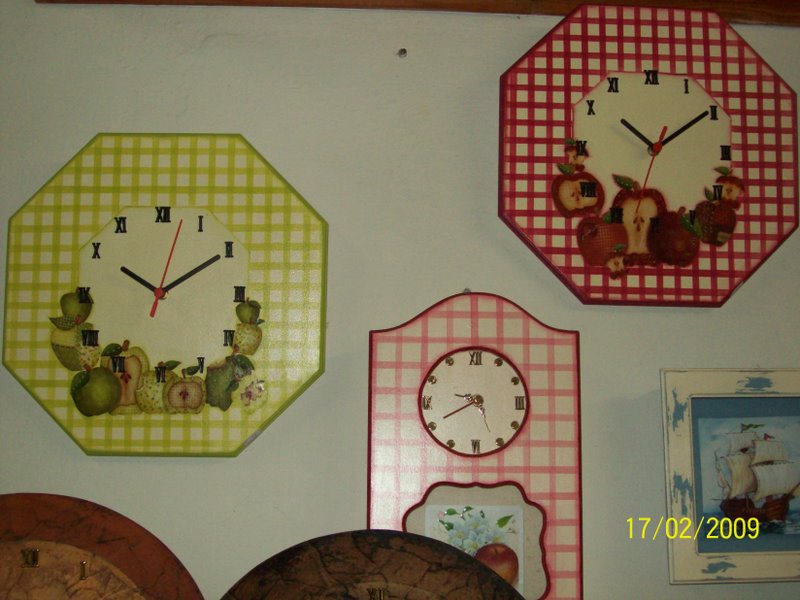This photograph, bearing the timestamp "17/02/2009" in the bottom right-hand corner as if taken from a camera, features a collection of uniquely designed clocks. In the top right-hand corner, a heptagonal clock adorned with Roman numerals displays a charming apple motif; these apples vary in depiction, showcasing whole apples, apples sliced in halves, and one distinctly bitten apple at the bottom of the clock face. This clock is further embellished with a grid pattern consisting of vertical lines.

On the left-hand side, a second heptagonal clock mirrors the design of the first but features green apples instead of red. Centrally positioned near the bottom of the photograph is another clock distinguished by its smaller circular frame, decorated with pink stripes. Below this clock, an image of an apple serves as a decorative feature.

Additionally, a picture of a sailboat can be observed hanging on the wall, adding a touch of nautical charm to the scene.